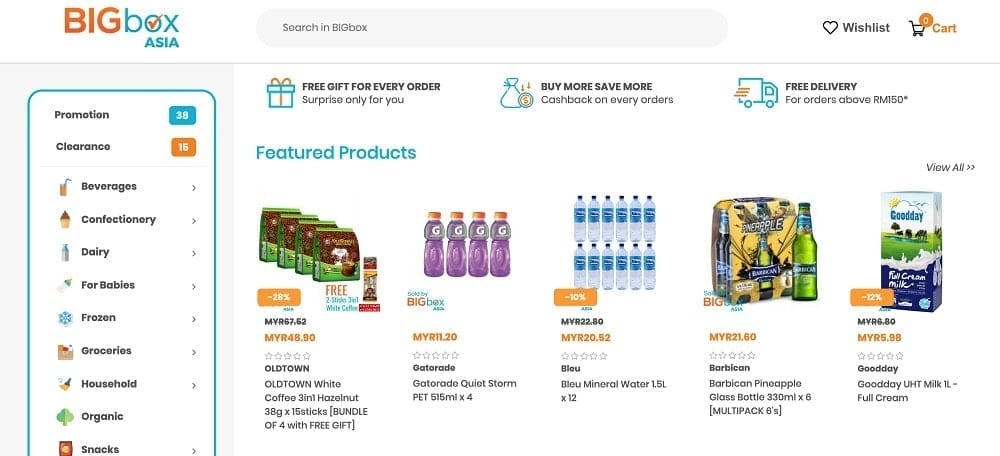In this image, we see a detailed screenshot of a website with a white background. In the upper left corner, there is bold orange text that says 'big' inside a blue text box, followed by 'Asia' in blue text. On the upper right, there is a gray text label 'Wishlist' accompanied by icons of a heart and a shopping cart.

Below this, on the left side, there is a vertical menu. At the top, the menu reads 'Promotion (38)' and 'Clearance (15)'. The menu continues with several categories, each represented with an icon. They include:

- Beverages
- Confectionery
- Dairy
- For Babies
- Frozen (represented by a snowflake icon)
- Groceries
- Household (represented by a broom icon)
- Organic
- Snacks

To the right of this menu, the image displays featured products. The first product is Old Town White Coffee priced at $48.90. To the right of it, there is an image of four bottles of purple Gatorade labeled 'Gatorade Quiet Storm, 4-pack.' Further to the right, there is an image of a 1.5-liter bottle of 'Blue Mineral Water.'